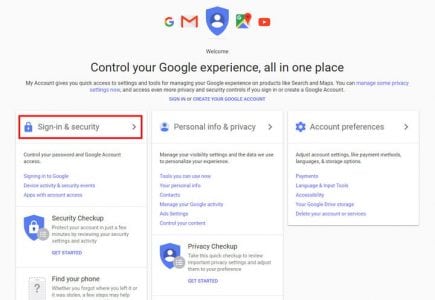The image displays the Google welcome page with a light gray background at the top. Prominently featured is the colorful Google logo, characterized by red, green, blue, and yellow letters. Adjacent to it is the Meta logo, distinguished by a stylized red "M". To the right of these logos is a blue badge with a black circle framing a simplistic white drawing of a head and square shoulders. Next, there is a green image marked with a red dot, though the details are unclear. On the far right is a red circle with a play button, likely representing YouTube.

Below the logos, a black banner reads, "Control your Google experience all in one place" in very small font. Further down, the page is sectioned into distinct boxes. The first box, labeled "Sign-in and Security," features a blue padlock icon and a red square framing the text written in blue. The lettering within this section is extremely small and difficult to read.

The next box, titled "Personal Info and Privacy," contains gray text with a faint gray arrow pointing to the right, accompanied by an icon depicting a circular head and square shoulders. Lastly, the section on the far right is labeled "Account Preferences" in gray text. It includes a blue circle with ridged edges and a gray arrow pointing to the right, although the lettering here is also quite faint and challenging to discern.